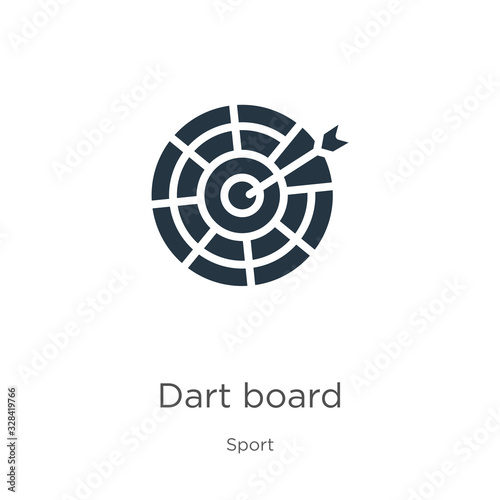This computer-generated image features a detailed dartboard consisting of four concentric rings, segmented appropriately, with an arrow piercing the bullseye at its center. The dartboard is blue, and the arrow has distinct blue feathers. Below the dartboard, the text "DARTBOARD" is displayed in a greyish font with a capital 'D', followed by the word "sport". Additionally, a vertical text on the bottom left reads "ADOBE STOCK" in black, alongside a divider and hashtag #328-419-766. The image has visible watermarks, including "ADOBE STOCK" in white text superimposed across the dartboard, indicating it's a stock photo available for purchase.